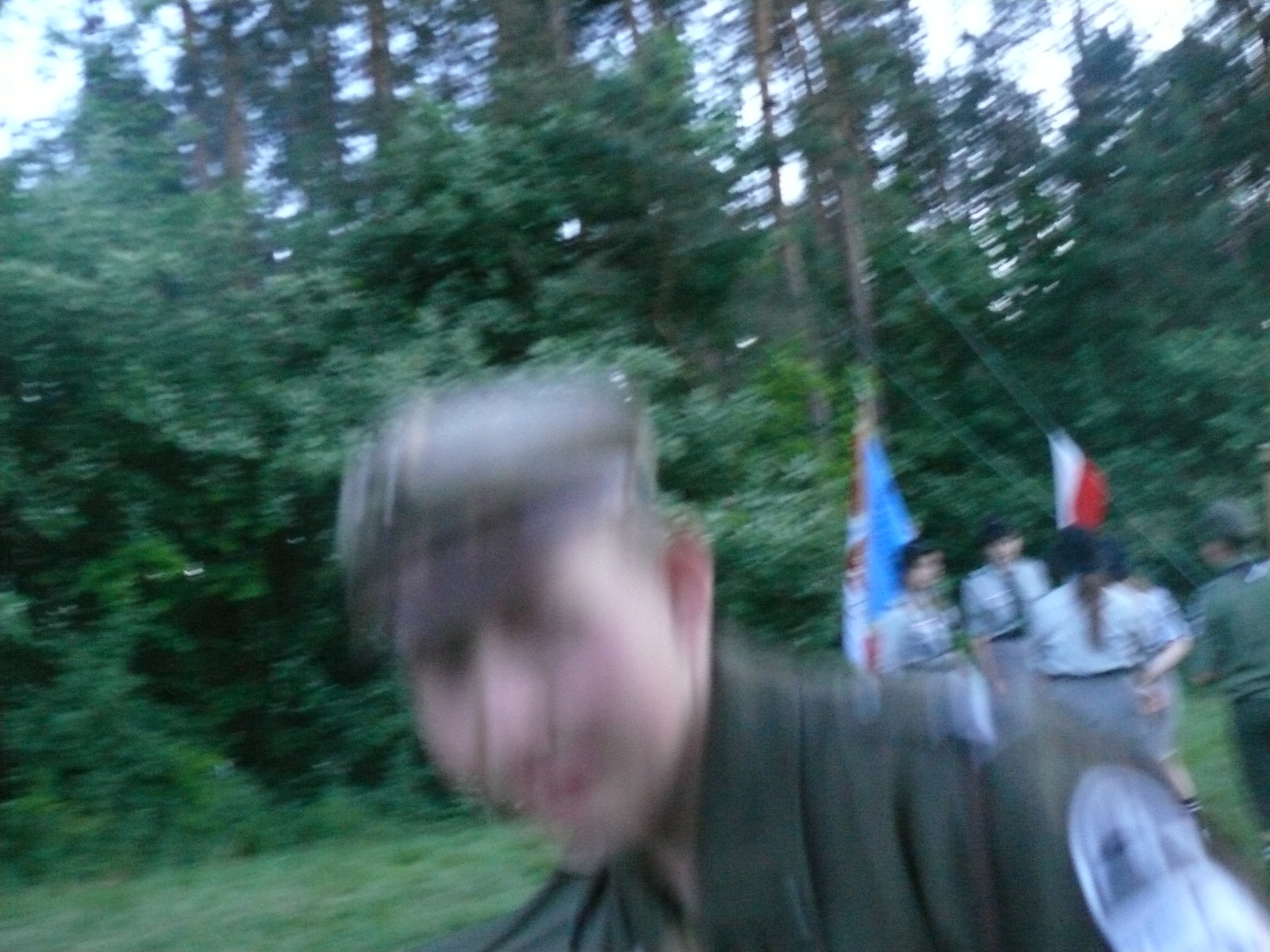In this captivating photograph, a group of individuals is gathered in a lush, natural setting, surrounded by dark green trees with prominent brown trunks. A sense of community and tradition is evident as they hang various flags, including one with a combination of blue, brown, and white, and another featuring white and red colors. The image is slightly distorted by a motion blur effect, giving it a dynamic, almost surreal quality.

At the foreground, a notable figure stands out, wearing a distinctive green hat with a brown brim and a matching green jacket. His facial features are indiscernible, adding a sense of mystery to his lighter skin tone. A black and white patch adorns his shoulder, hinting at an affiliation or role within the group.

In the background, a similarly dressed individual in a green outfit can be seen alongside three others in gray shirts, one of whom sports a tie. These three are also dressed in gray skirts and appear to be wearing blue hats, suggesting a uniform or coordinated attire. The scene captures a moment of camaraderie and teamwork amidst the vibrant embrace of nature.